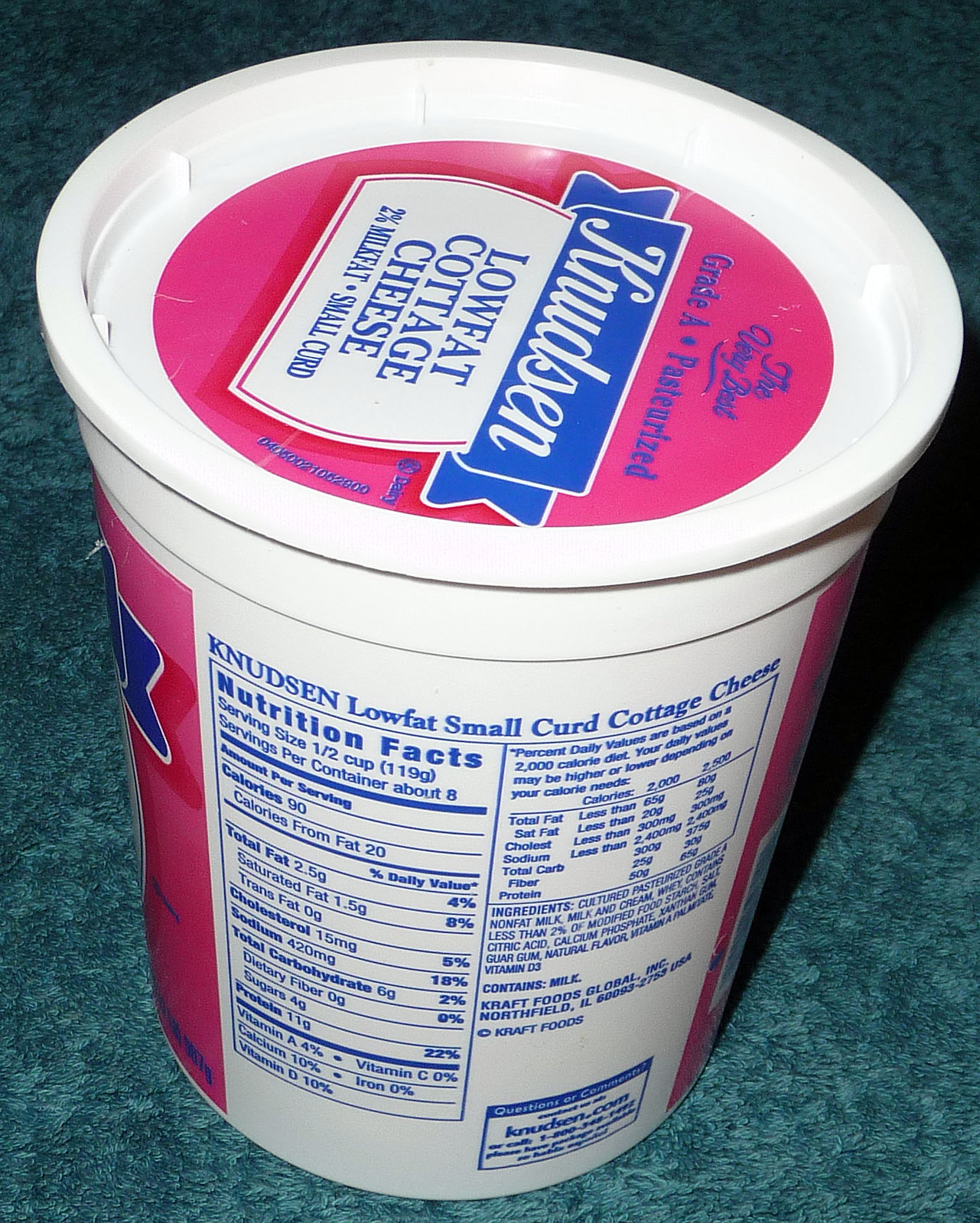This detailed photograph captures a white plastic container of Knudsen Low-Fat Small Curd Cottage Cheese prominently placed on a turquoise marble-like tabletop. The container features a vibrant pink and blue label. On the top of the white lid, a round pink label boasts the brand name "Knudsen" in a blue ribbon-like pattern, and directly below in a white square, the product description states "Low-Fat Cottage Cheese, 2% Milk Fat, Small Curd." Viewing the side of the container, the Nutrition Facts label is prominently displayed, revealing details about the serving size, calories, and nutritional content in blue text. The label also provides an ingredient list, confirms that the product is Grade A pasteurized, and mentions it is manufactured by Kraft Foods in Illinois.